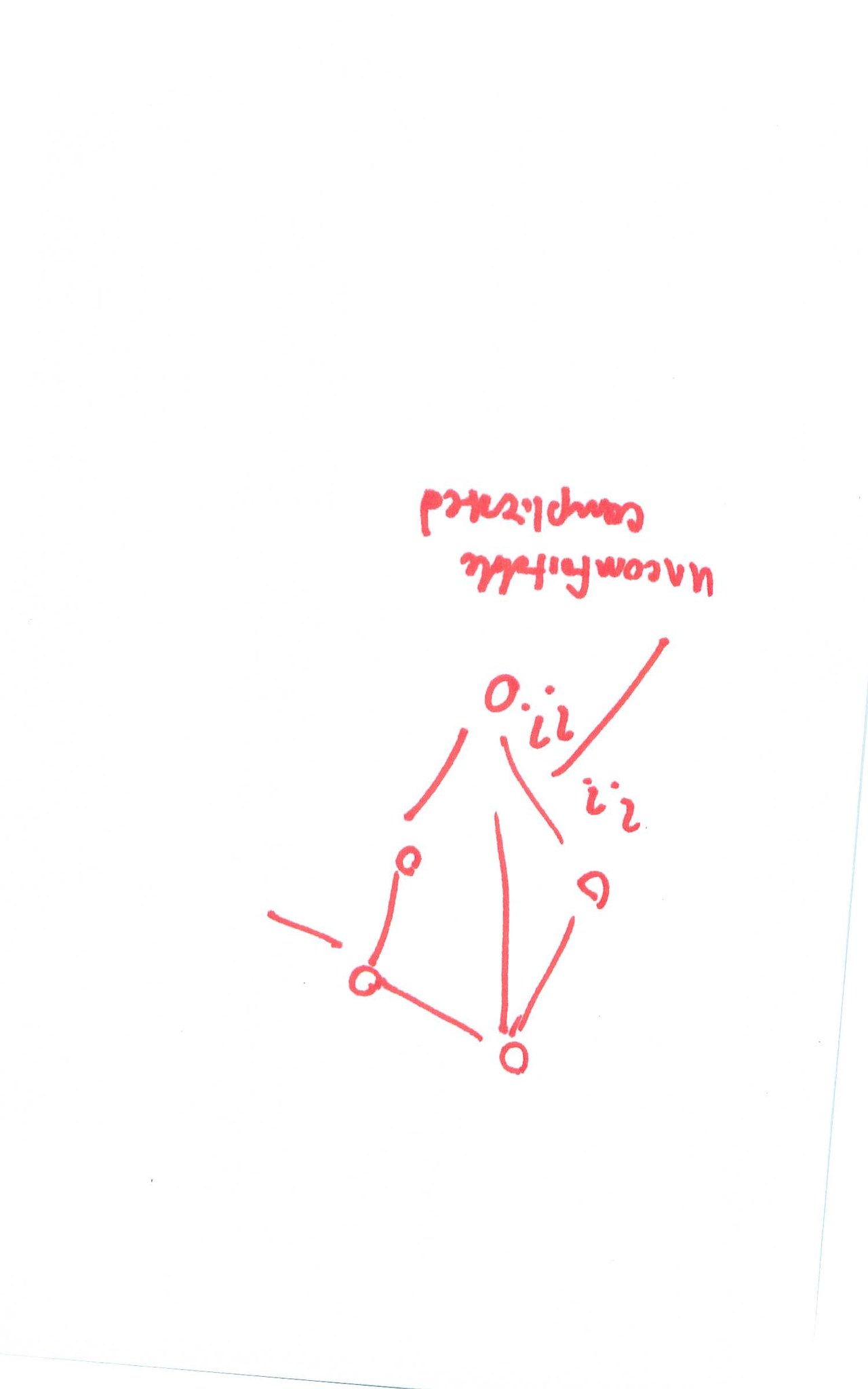The image features a scrap of paper that appears to be an intricate diagram drawn using a red marker. The diagram consists of lines connecting small circular shapes, resembling a schematic of a chemical composition or molecular structure. The note is oriented upside down, and at the top, there is a segment of text that includes the words "complicated" and "uncomfortable." This text seems to be referencing a bond illustrated between two atoms or molecules within the diagram. Additionally, question marks flank the line pointing to this particular bond, indicating uncertainty or inquiry. The diagram itself includes a total of five small circles connected by six lines, all meticulously drawn in red marker.